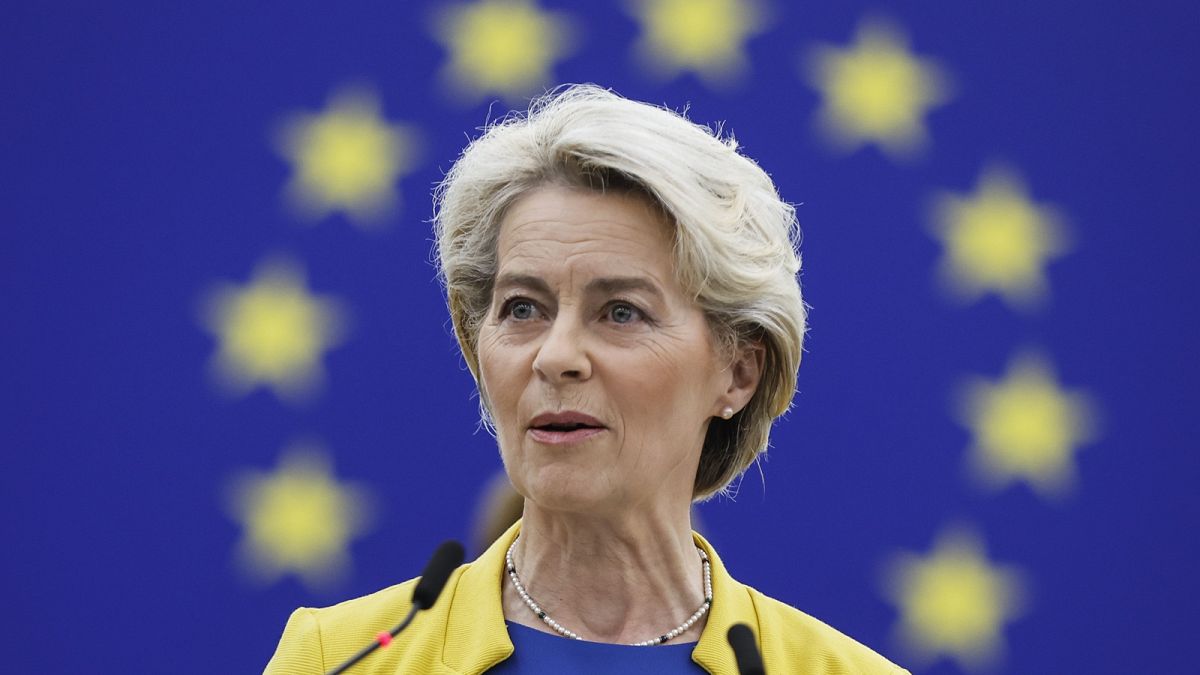The image is a photograph of Ursula von der Leyen, the current President of the European Commission, who appears to be giving a speech. She is depicted with her neatly styled, controlled blond hair, indicative of her political presence. von der Leyen is adorned in a yellow jacket over what seems to be a blue top, and she is wearing a necklace, possibly made of pearls or beads. In front of her are two small black microphones, emphasizing her engagement in speaking to an audience. The backdrop features the European Union flag, distinguished by its blue background and circle of yellow five-pointed stars, although slightly out of focus.